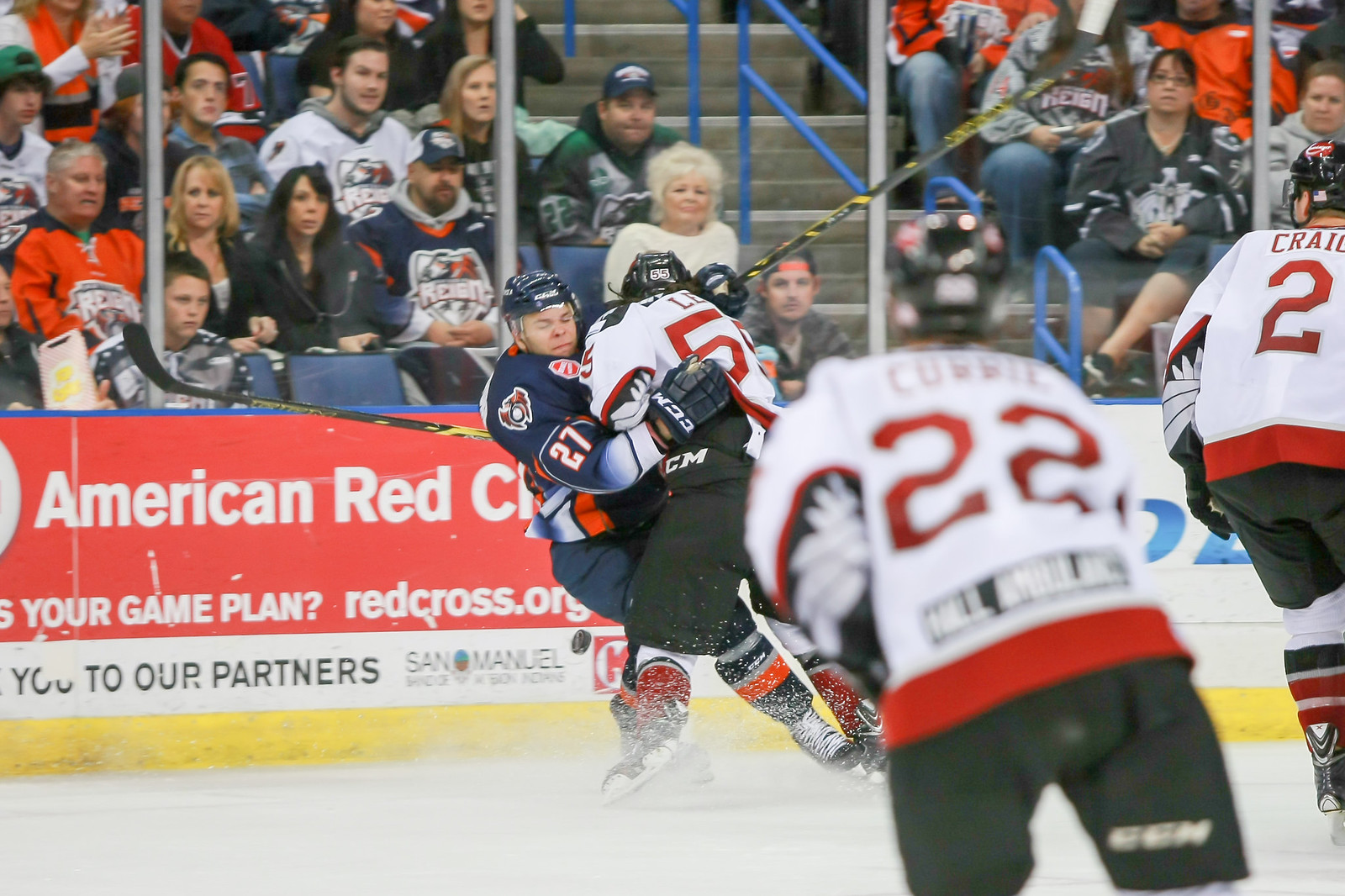The photograph captures a thrilling moment in an ice hockey game, possibly professional or semi-pro, with a packed stadium full of spectators behind the glass barrier. Central to the scene are two players in mid-collision: one in a navy blue jersey with the number 27, who is falling backward, and another in a white jersey with red accents, including the number 5, who appears to be tackling him. The action has scattered ice beneath them, and their sticks are raised in the air. Flanking the scuffle are two other players from the team in white jerseys, numbers 22 and 2. The arena features prominent advertisements, including one for the American Red Cross with "American Red" and "redcross.org" visible, as well as another ad mentioning "San Manuel." The crowd of spectators intensely watches the unfolding drama on the rink. The white jerseys also sport black and red stripes on the sleeves and bottom, completing the detailed ensemble of the players.